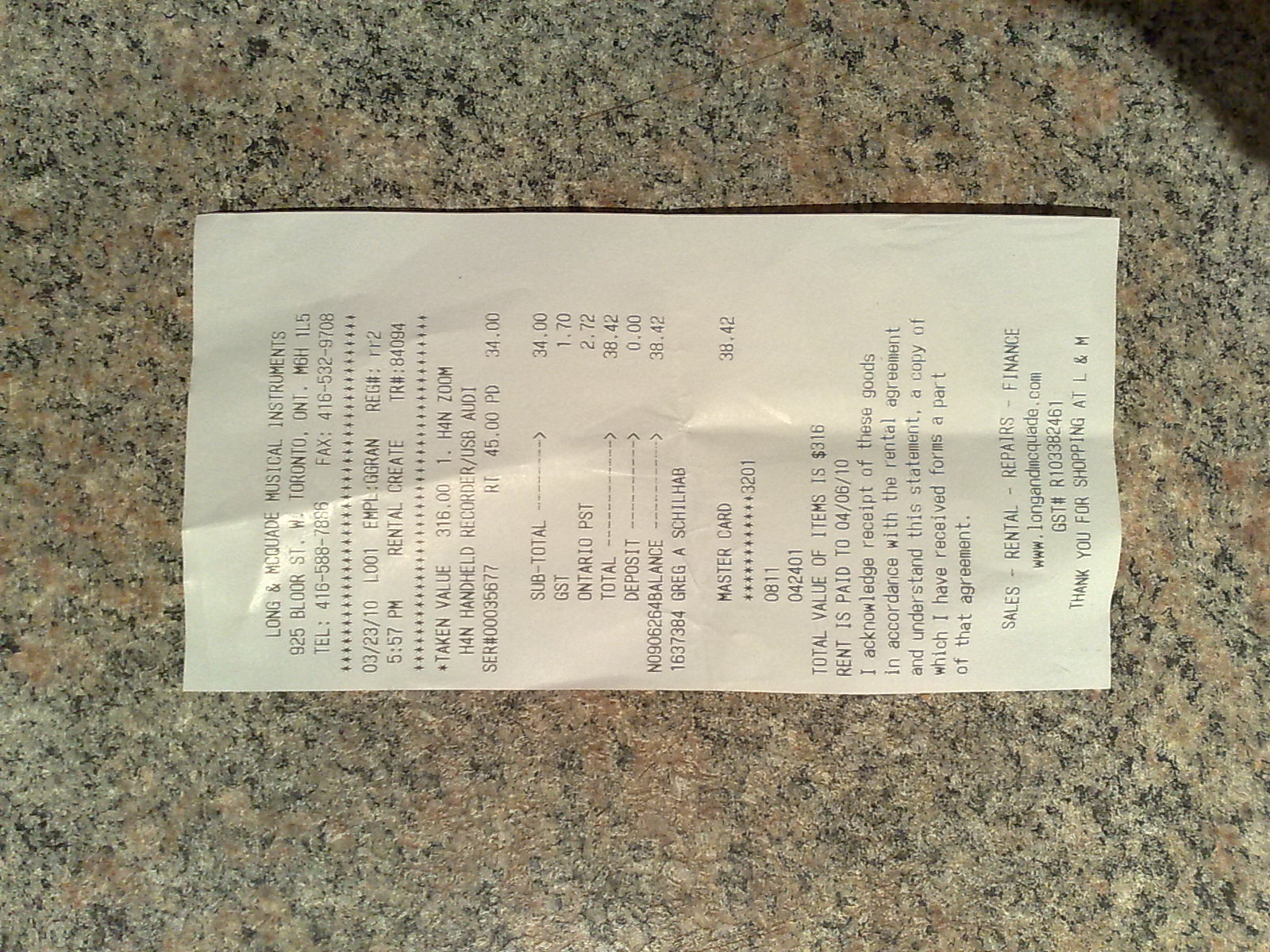On a textured, pebbled walkway, there lies a framed receipt from a musical instrument store, dated March 23, 2010, at 5:57 PM. The receipt details the rental of a handheld recorder, valued at $316.00. The initial rental charge for the device was $34.00, with additional taxes bringing the total to $38.42. The payment was processed via MasterCard. The receipt also states that the recorder must be returned by April 6, 2010, and includes a signed acknowledgment of the rental agreement.